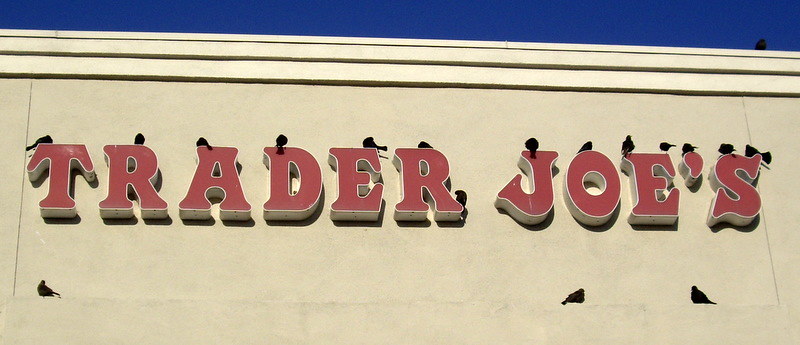In this striking image, the prominently displayed Trader Joe's sign adorns the exterior of one of their storefronts. The iconic red letters, trademark colors of the brand, are evenly spaced and crisply defined. Adding a whimsical element to the scene, several birds perch atop the letters. On the word "Trader," each letter hosts its own avian visitor, with an additional bird hanging off the "R." Moving to the words "Joe's," a bird is perched on the "J," "O," and two on the "E." Additionally, one bird sits on the apostrophe, and two birds rest on the "S." Completing the lively tableau, three birds casually hang out on the ledge just below the Trader Joe's sign, lending a unique, natural charm to the storefront.